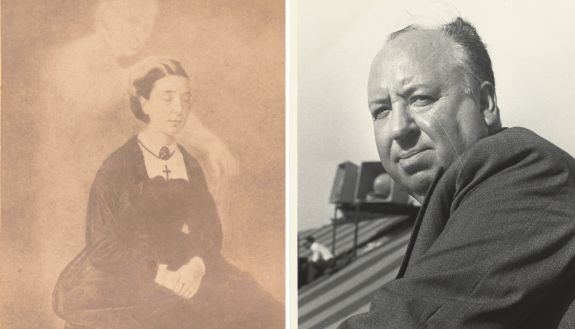In these combined images, the left picture features an ethereal, almost smoky depiction of a woman in old-fashioned Victorian attire, characterized by her black dress and white undershirt. She is adorned with a cross necklace and has her eyes closed, hands folded, evoking a serene, contemplative posture. Behind her, a ghostly figure of an old man with a raised hand touching the back of her head adds an eerie, spectral quality to the scene. The image radiates a vintage, mysterious ambiance. 

Conversely, the right picture presents a clear, black-and-white photograph of an older Caucasian man who bears a resemblance to Alfred Hitchcock. He appears to be slightly balding and is positioned outdoors. In the background, there is a rooftop with another man sitting on the left side, possibly on elevated stands like bleachers, indicated by the visible sky and surrounding environment. The juxtaposition of these two images blends the enigmatic past with a clear moment from mid-20th century life.